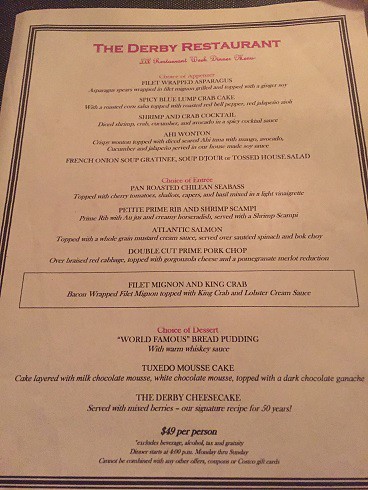The image depicts a white menu with a bold black border. At the top, the heading "The Derby Restaurant" is written in either red or pink font. Directly below, there is additional text in cursive that is somewhat difficult to decipher, with the first word appearing to be "Lil."

The main body of the menu lists various dishes. The first few items, which are relatively easy to read, include:

- Fillet Wrapped Asparagus
- Spicy Blue Lump Crab Cake
- Shrimp and Crab Cocktail

Following these items, there are several more difficult-to-read dishes including types of wontons. 

The menu proceeds with a section labeled "Choice of Entrée" featuring:

- Pan-Roasted Chili Beans
- Sea Bass
- Petite Prime Rib and Shrimp Scampi
- Atlantic Salmon
- Double Cut Prime Pork Chop
- Fillet Mignon and King Crab

Next, the menu provides dessert options with detailed descriptions:

- World-Famous Bread Pudding with Warm Whiskey Sauce
- Tuxedo Mousse Cake, layered with milk chocolate mousse and white chocolate mousse topped with dark chocolate ganache
- Derby Cheesecake served with mixed berries, noted to be a signature recipe for 50 years

At the very bottom of the menu, it states "$49 per person" along with another line of text that is difficult to read.